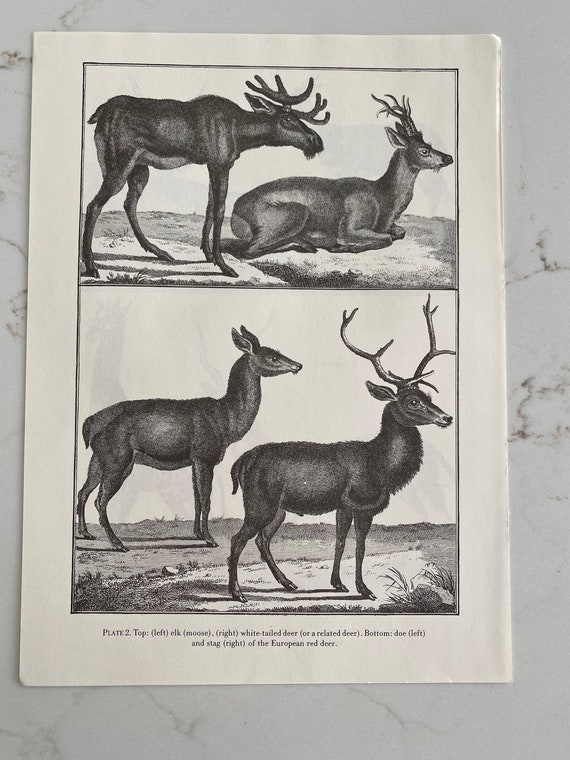A black-and-white sketched illustration taken from a book is set against a white marble surface, speckled with black flecks. The page displays four distinct animals, each identified by captions beneath them. The top left features a fully-shaded moose labeled “elk moose,” while to its right, a lighter-shaded, reclining animal is identified as a "white-tailed deer or related deer." On the bottom left, an upright doe labeled "bottom doe" stands clearly, and next to it, a dark-shaded stag with prominent antlers is marked as "stag of the European red deer." The detailed sketches and inscriptions provide a clear depiction of each animal and their respective species.